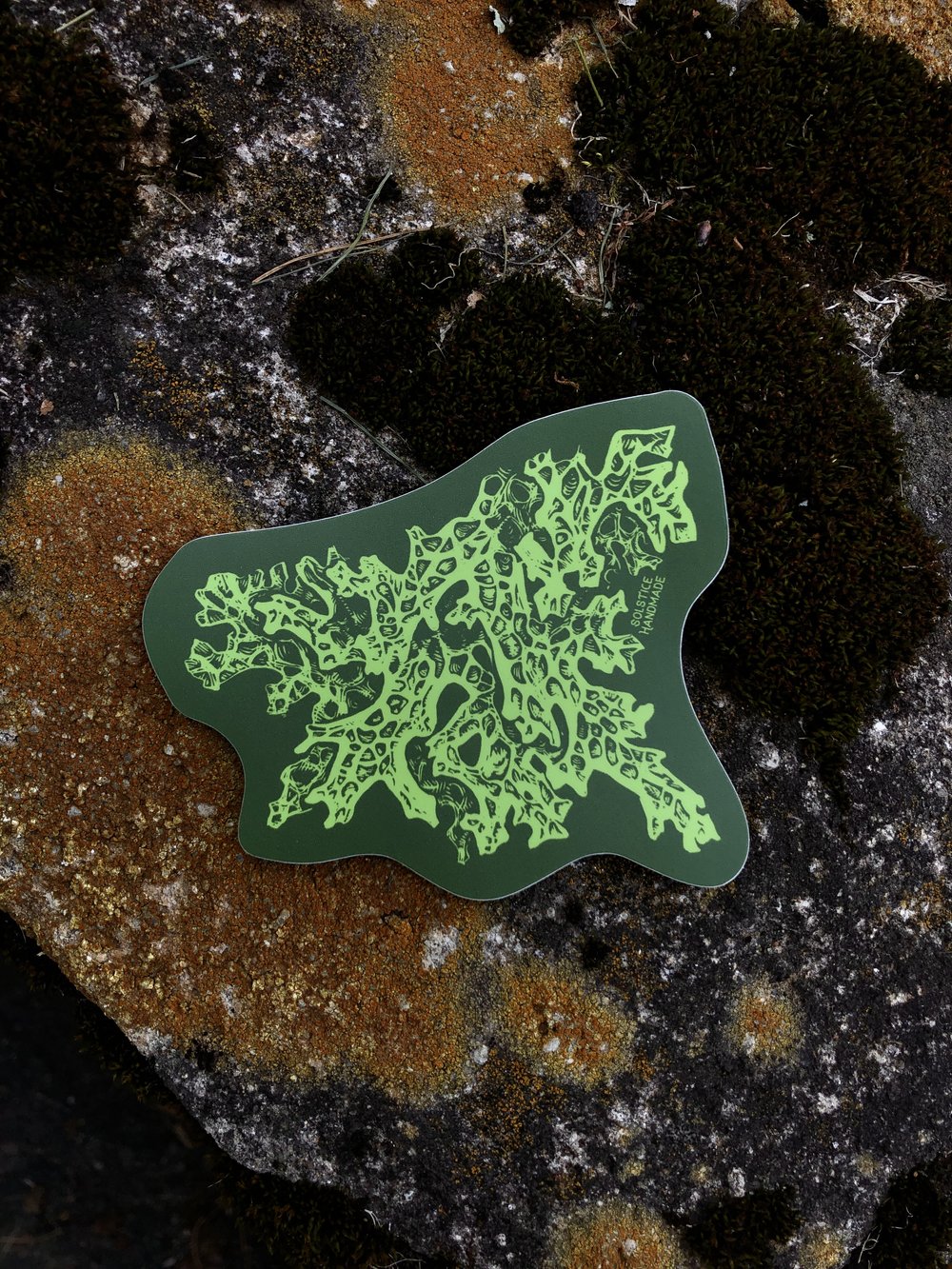In the image, a green sticker or logo labeled "Solstice Handmade" is prominently displayed, dropped on a ground that is primarily black with white speckles, reminiscent of snow. The green sticker, shaped somewhat like algae or a tree with intricate, web-like extensions, has a detailed design with smaller, lighter green filaments branching out. The ground also features large brown patches that resemble moss or weathered rock, creating a textured, uneven surface. This juxtaposition of the green sticker against the dark, speckled, and brown-streaked background gives the image a distinct topographical feel, as if viewed from an aerial perspective.